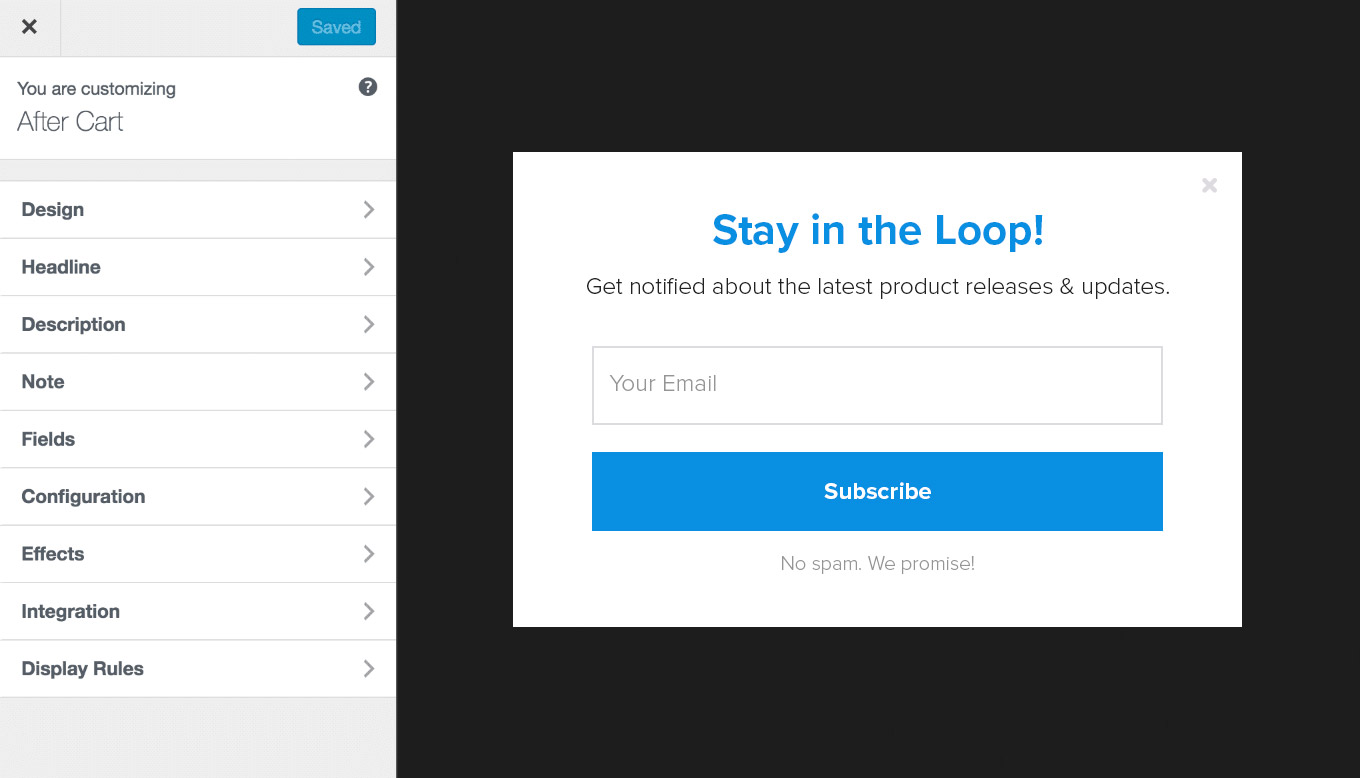This image depicts a screenshot of a website or computer interface featuring a pop-up subscription form on the right-hand side. The main focal point is a large black rectangle containing a smaller white rectangle with a light gray X icon in the top right corner. Within the white rectangle, the text "Stay in the loop" is highlighted in blue font. Below this headline, the message "Get notified about the latest product releases and updates." is clearly displayed.

Beneath the message is a light gray-outlined rectangle labeled "Your email," followed by a solid blue button with white lettering that reads "Subscribe." Further down, a gray text assures, "No spam. We promise!"

To the sides of the pop-up, a large X icon is available for closing the section. Above the pop-up, another rectangle reads "Saved" and indicates the user is in the process of "customizing after cart." A sequence of clickable words, each accompanied by an arrow, lists options including "Design," "Headline," "Description," "Note," "Fields," "Configuration," "Effects," "Integration," and "Display rules."